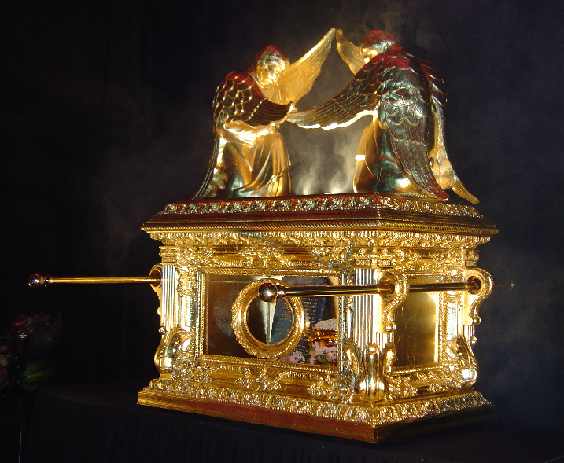This image, likely taken in a museum, showcases an ornate, historical artifact set against a dark black and gray backdrop. The centerpiece is an opulent litter, covered entirely in gold leaf, featuring an intricate design of carved gilt embellishments. The litter boasts cut-out windows and prominent handles on either side, hinting at its use in classical times to transport royalty, much like Cleopatra, by bearers. 

The structure exhibits a dark red-brown wooden base and an elaborately decorated upper section with gold medallion trims and vertical column-like accents. Distinctively, the litter is adorned with two large, sculpted figures on top. These figures, possibly griffins or sphinxes, are richly detailed and appear to be engaged in a dynamic pose, somewhat resembling wrestlers with arms extended towards each other. 

The statues are draped in garments with red, gray, and gold highlights and feature darkened wings, further enhancing the regality of the artifact. There is also an additional gold rod with a black ball at its end protruding from the side of the litter, adding to the intricate details. Overall, this splendid, gold leaf-covered ornament exudes a sense of grandeur and historical significance.